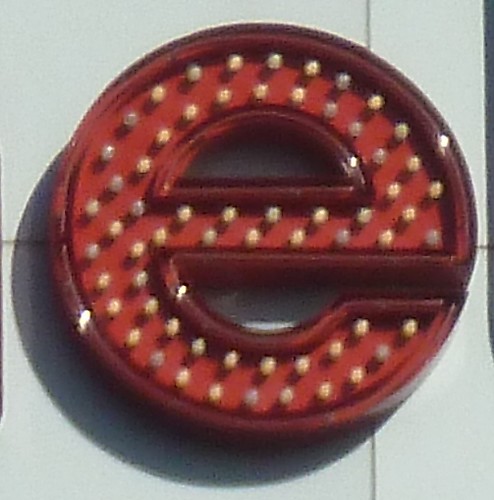This photograph captures a large, decorative, lowercase letter 'e' mounted on a wall. The 'e' is nearly circular in shape with a cutout top half, transitioning into an open right side to form its distinctive shape. Boldly colored in red with a darker red, almost burgundy border, the letter 'e' features an array of light bulb-like dots inside, varying between bright yellow and silver-gray, hinting that it may illuminate at night. The mounting surface appears to be a white wall, possibly tiled, with an intersection of tiles or stripes slightly obscured by the letter's right side. Natural sunlight casts a shadow from the top right to the lower left, indicating the photograph was taken during the day, possibly suggesting the sign's installation outside a store.